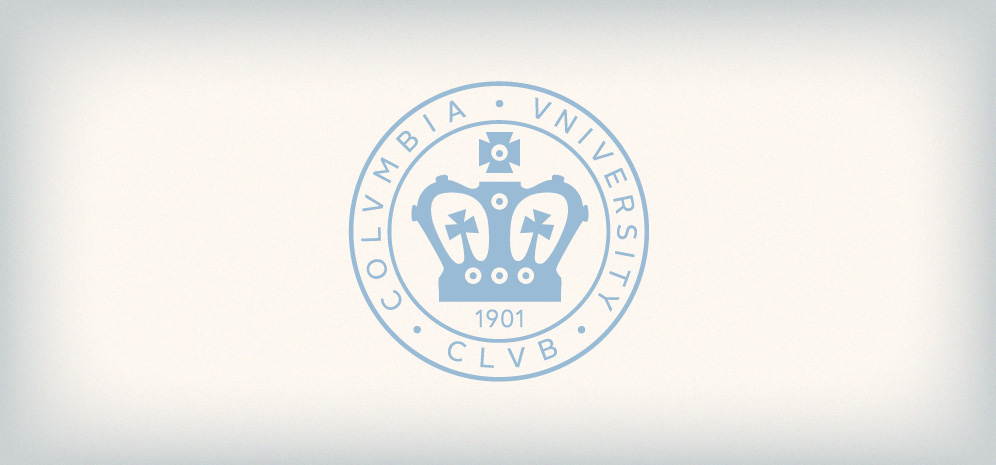This detailed image features a cropped, horizontal rectangular logo of the Columbia University Club from 1901. The background of the image blends from white in the center to a faded medium gray along the edges, giving it a subtle, framed appearance. 

At the heart of this rectangular image is a circular logo, which itself contains two concentric circles. Between these circles, the name "ColVmbia.Vniversity.ClVb" is inscribed, notably using the letter "V" in place of the traditional "U". Small dots separate each word, enhancing the classic aesthetic of the design. 

Within the inner circle, a stately crown takes center stage. This crown features two open areas, each with a small cross, and a total of four crosses in and above the crown. Small white circles adorn the bottom of the crown, three at the base and one placed centrally between the two crosses. Directly beneath this emblematic crown, the year "1901" is prominently displayed, anchoring the historic and distinguished look of the logo. The entire composition sits against a cream-colored background, which, together with the gray borders, adds to the aged, elegant feel of the image.